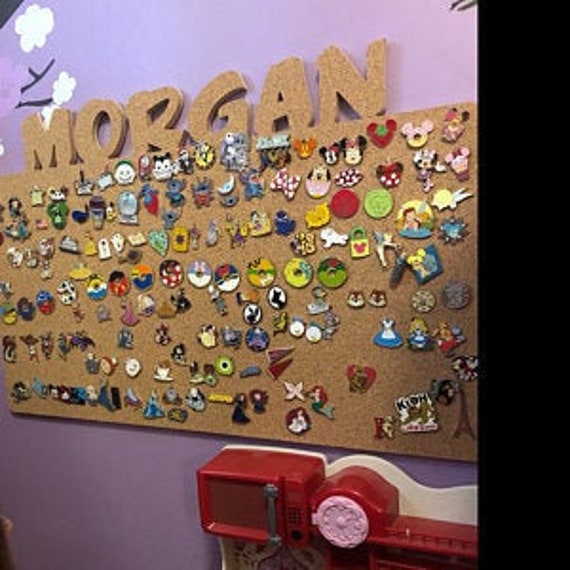The photograph captures an indoor scene with a square, 4x4 inch frame. Dominating the image is a purple wall adorned with a brown corkboard centered on it. The corkboard measures approximately 2 inches in height and features the name "Morgan" spelled out in matching corkboard material at the top. The upper left corner of the purple wall is decorated with painted white clouds, black branches, and what appears to be a light purple mouse head. The corkboard hosts a vast collection of various pins and buttons, including recognizable characters like Mickey and Minnie Mouse, Pluto, Donald Duck, and the Little Mermaid, although many are too small or blurry to definitively identify. The bottom right corner of the image reveals a red, plastic children's toy resembling a microwave, situated near what seems to be a play kitchen area. The photograph has a solid black border running from the top right corner down to the center of the right edge.